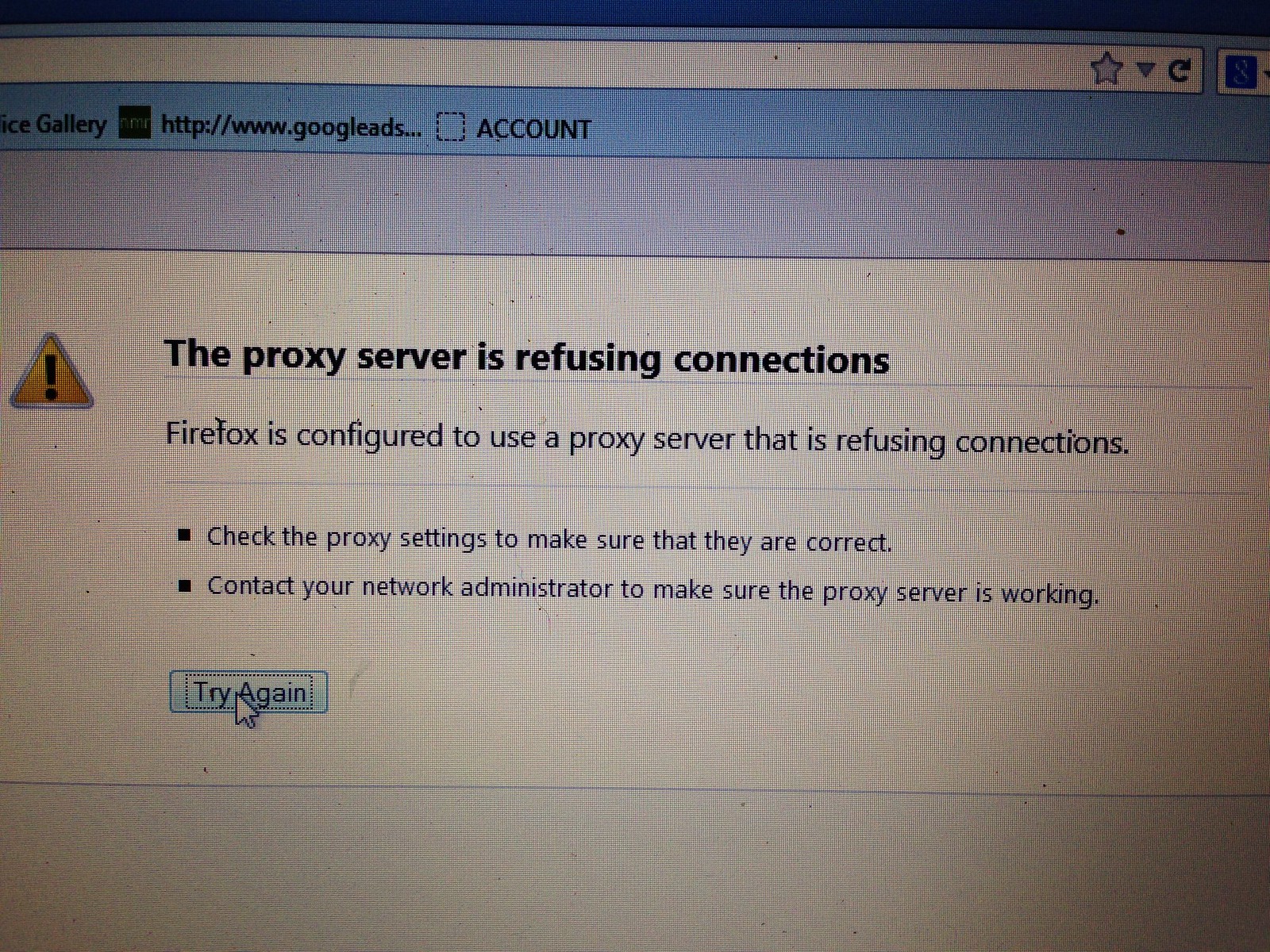In this detailed image, we observe a computer screen displaying a Firefox browser window, which prominently features a warning message that reads, "The proxy server is refusing connections." This issue arises because Firefox is configured to use a proxy server that is currently rejecting connections. The primary text is centered and clearly visible, with an accompanying yellow warning triangle containing a black exclamation mark situated to its left.

Below the warning message, the browser suggests two potential solutions: first, to check the proxy settings to ensure their accuracy; and second, to contact the network administrator to confirm the proxy server's functionality. Further down, there is a rectangular button labeled "Try Again," highlighted in turquoise, with the mouse cursor hovering over it. The 'T' in "Try" and the first 'A' in "Again" are capitalized.

Additionally, the top portion of the browser displays a bookmarks toolbar, where one bookmark is partially labeled as "google leads..." and another is titled "account." The address bar is empty, and a gray banner spans horizontally beneath the bookmarks.

Overall, the image captures a moment of technical troubleshooting within the Firefox browser, emphasizing the detailed error message and suggested actions while visually situating elements like the cursor, warning icon, and bookmarks for comprehensive context.